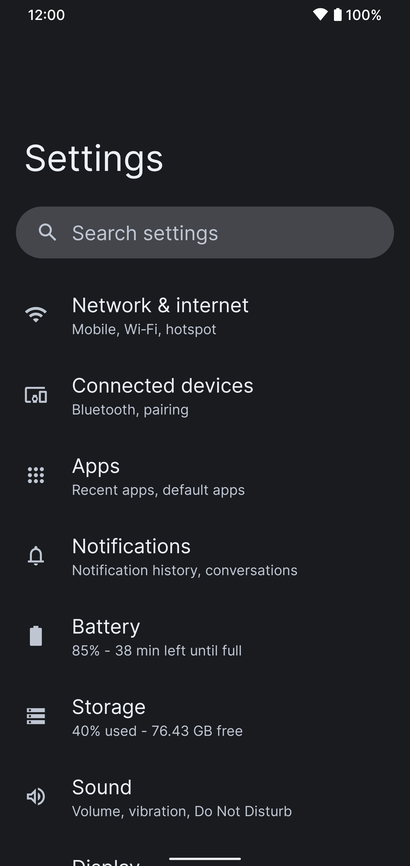This image is a screenshot from a smartphone displaying the settings menu at 12:00 PM with a fully charged battery at 100%. The background is black, enhancing the clarity of the dark gray "Settings" header at the top. Below the header is a search bar, also dark gray with a magnifying glass icon, labeled "Search settings."

The settings menu is organized into several categories:

1. **Network & Internet:**
   - Sub-options: Mobile, Wi-Fi, Hotspot

2. **Connected Devices:**
   - Sub-options: Bluetooth, Pairing

3. **Apps:**
   - Sub-options: Recent Apps, Default Apps

4. **Notifications:**
   - Sub-options: Notification History, Conversations

5. **Battery:**
   - Status: 85% charged, with 38 minutes left until fully charged

6. **Storage:**
   - Status: 40% of storage used, 76.43 GB free

7. **Sound:**
   - Sub-options: Volume, Vibration, Do Not Disturb
   - Icon: A speaker with sound waves emanating from it

8. **Display:** 

Icons representing each category are situated to the left of their respective labels, visually indicating their functions, such as a speaker icon for the sound settings. This screenshot captures all the essential elements of the phone's settings interface in detailed clarity.